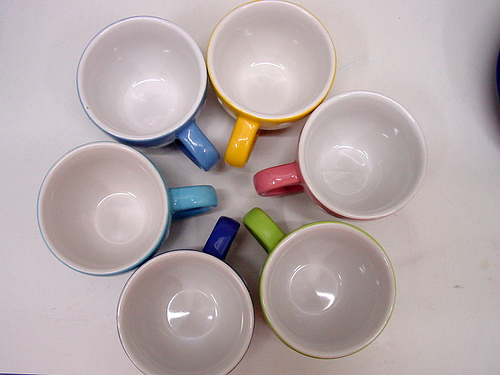This is a detailed colour photograph taken from an aerial, bird's-eye view, showcasing six ceramic mugs arranged in a circle on an off-white, possibly untextured surface. The mugs' handles are turned inward, forming a smaller circle within the larger one. Each mug has a white interior and a brightly coloured handle, which are also partially visible on the outer rims. The colours of the mug handles, starting from the top left in a clockwise direction, are medium blue, yellow, coral-pink, bright green, dark blue, and a lighter, powder blue. Light reflects softly off the shiny, clean surfaces of the mugs, adding a slight glow to the scene. There are subtle shadows towards the upper left and a tiny black speck or flaw visible on the powder blue mug. Additionally, a small black line and an out-of-focus shadow can be seen on the background near the bottom left and the top right corners, respectively. The composition gives an almost floral impression, making the simple arrangement visually engaging.